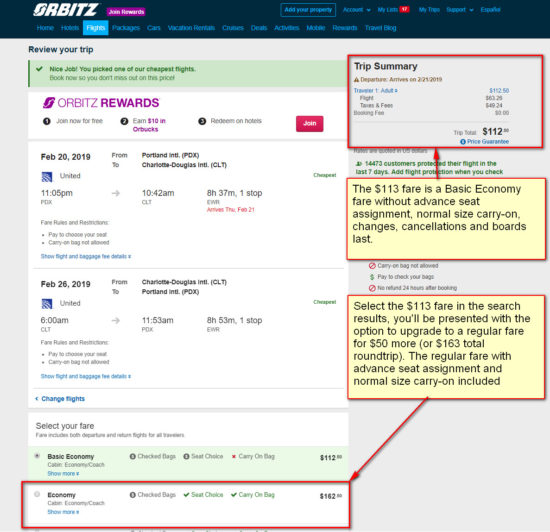The image depicts a detailed view of the Orbitz website, specifically focusing on booking flights. The main content area shows a trip summary and a call-to-action for booking. At the top right corner, the "Trip Summary" section highlights the following:

- One adult airfare: $112.50
- Flight cost: $63.25
- Taxes and fees: $49.24
- Booking fee: $0.00
- Total trip cost: $112.50

This section is emphasized with a red border. Below the summary, a yellow box, also circled in red, informs travelers that the $113 fare is a basic economy option. This fare does not include an advanced seat assignment but allows for a normal-sized carry-on. Additional restrictions include limited changes, cancellations, and boarding last.

The website suggests that if you select this $113 basic economy fare in the search results, you can upgrade to a regular fare for an additional $50, making the total $163. This regular fare includes an advanced seat assignment and a normal-sized carry-on bag.

On the left side of the image, flight details are displayed, though not highlighted in red. It shows a roundtrip itinerary with the following specifics:
- Departure date: February 20th, 2019
- From: Portland International Airport (PDX)
- To: Charlotte Douglas International Airport (CLT)

Overall, the image conveys options for booking an economical trip with additional details for upgrades and specific flight information.